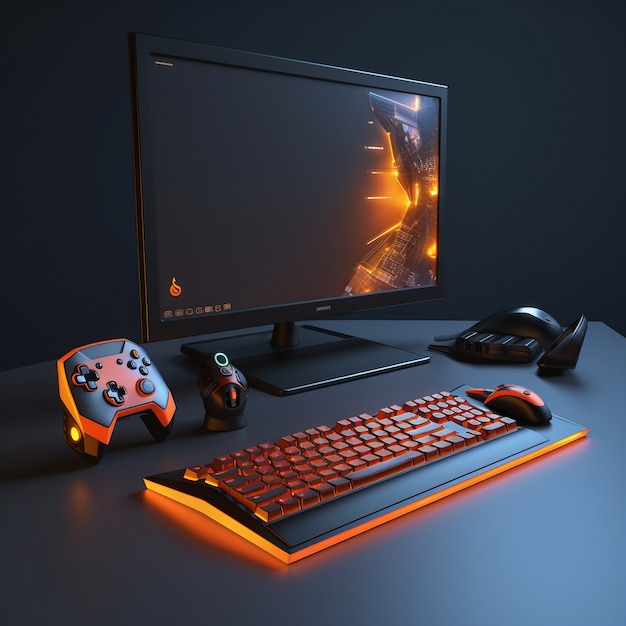The image displays a detailed gaming setup positioned on a sleek black table. At the center of the setup is a desktop monitor, also black, with a dark screen that dominates the top half of the image. In front of the monitor, a black keyboard with a subtle orange glow is placed at a 45-degree angle, roughly in the center-bottom area. To the right of the keyboard lies a black mouse with an orange top, and below the keyboard sits another mouse. Positioned to the upper left of the keyboard is a peculiar silver game controller, emitting an orange light, and nearby is a small, indistinct, black device with a blue ring, resembling a webcam. The entire arrangement is enveloped in a dark theme with sporadic orange highlights, contributing to the immersive feel of a sophisticated gaming environment.